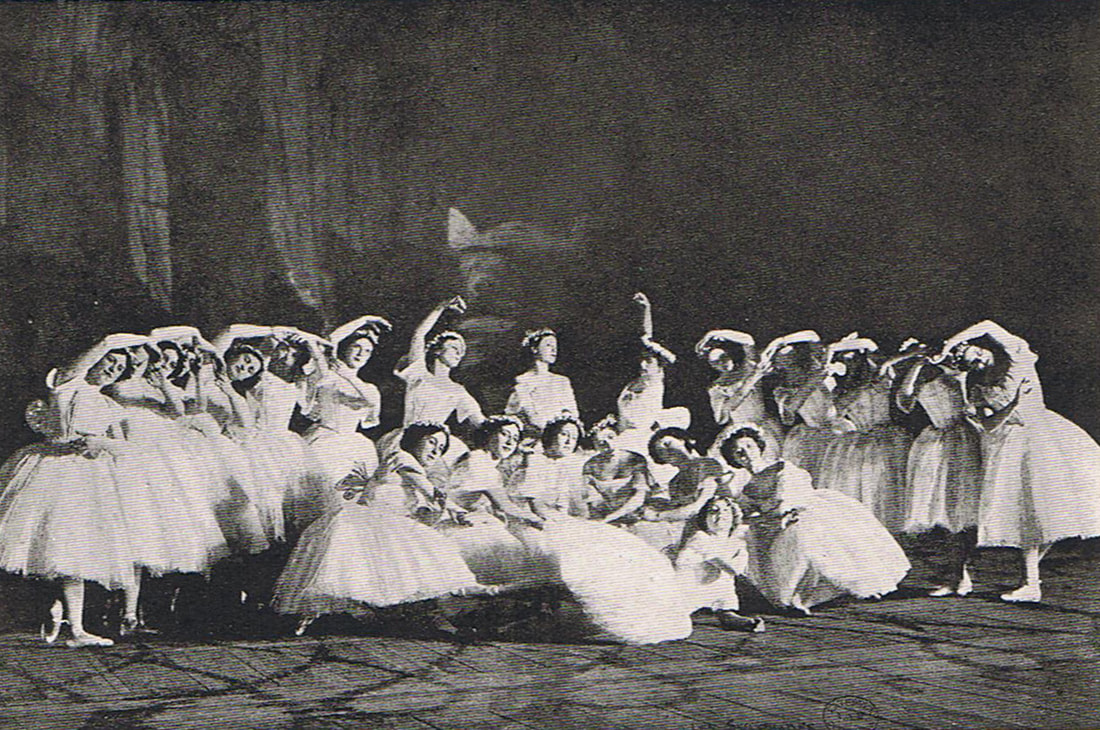This black-and-white, grainy photograph captures a choreographed group of women, likely ballerinas of European descent, posing gracefully on a dimly lit stage. The performers are arranged in two distinct half-circles. In the foreground, the women are crouched and leaning inwards, creating an intimate, interconnected formation. Behind them, a row of dancers stands with arms elegantly arched overhead, tilting towards the center. At the heart of the formation, a single dancer stands with her arms down by her sides. All the performers are dressed in matching white dresses adorned with large plumes at the bottom, complemented by white floral headpieces. This meticulously arranged scene is a striking representation of ballet artistry.